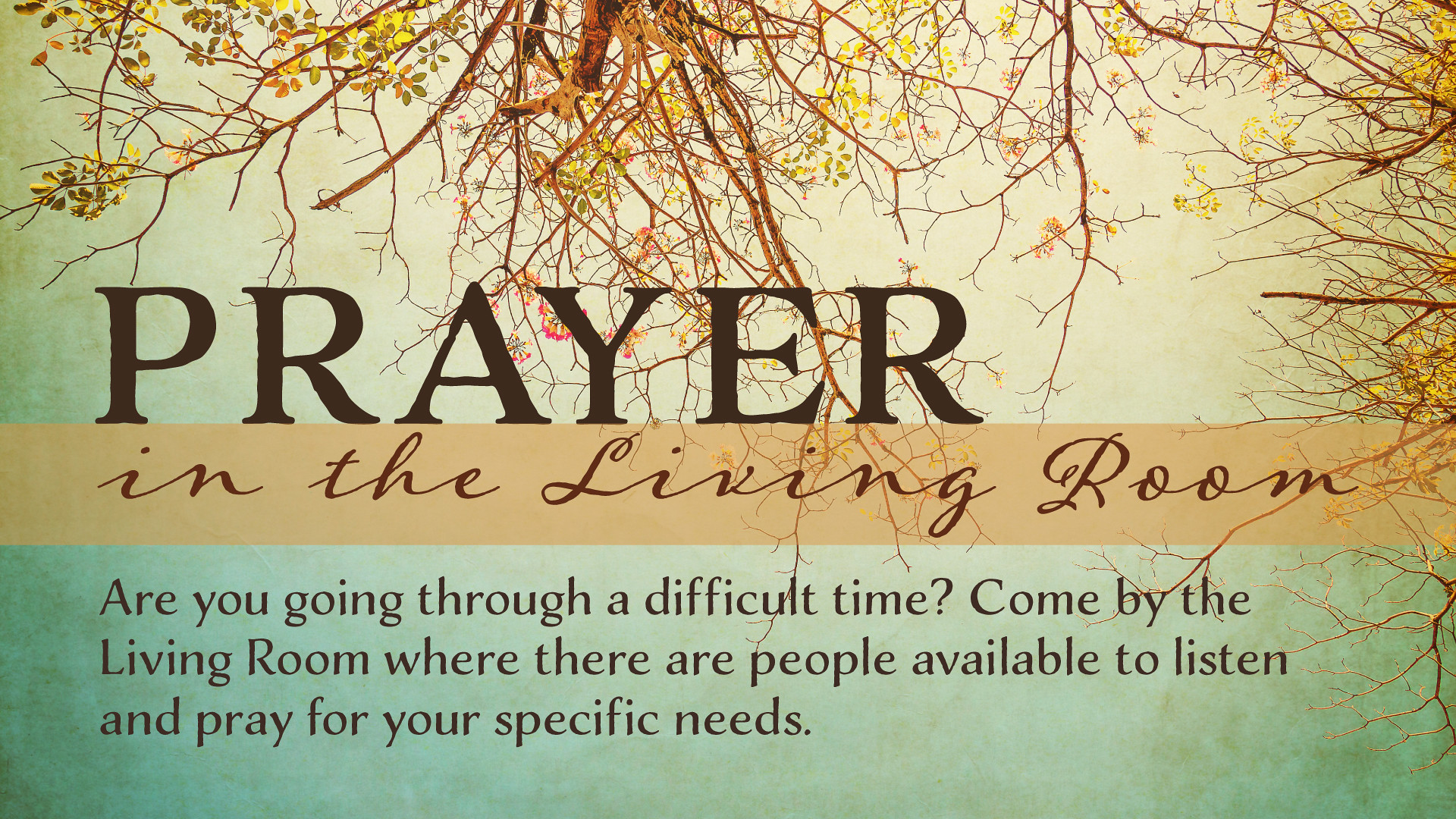The image features a graphic commonly shared on social media, resembling a postcard, article, or greeting card. The background transitions from a light blue gradient at the bottom to a yellow gradient at the top. At the top, dark brown tree branches with minimal green, yellow, and brown leaves can be seen, possibly giving the appearance of looking up from under a tree.

In the center, the word "Prayer" is prominently displayed in a large serif font, colored dark brown. This is flanked by additional text encapsulated in a small rectangular box that reads "in the Living Room" in a script or handwritten font, also dark brown. Below, a smaller dark brown text invites those experiencing difficult times to come by the living room, where people are available to listen and pray for their specific needs.

The overall design includes hues of off-green, teal, peach, brown, and gold, adding warmth and a sense of comfort. The layout and style suggest a heartfelt marketing message intended to provide support and solace to those in need.